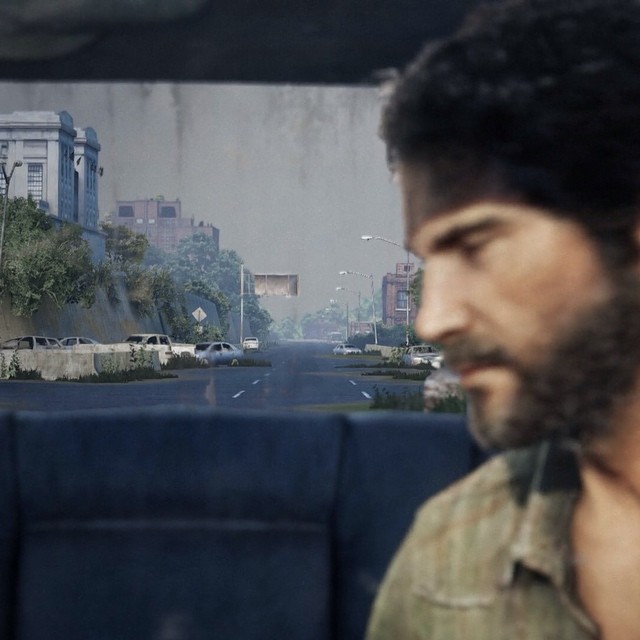In this color screenshot from the acclaimed video game series "The Last of Us," we are presented with a detailed view of the backseat of a vehicle. The seats, upholstered in dark blue fabric, constitute much of the immediate context. Positioned prominently on the right side of the image, we see the protagonist, Joel Miller. He is captured in profile facing left, with his eyes gently closed. 

Joel, depicted as a middle-aged man with short dark hair and a full beard, is attired in a brownish-gray button-down shirt equipped with a collar. The texture and folds of his shirt are subtly illuminated, adding a layer of realism to the depiction. His facial expression is serene and peaceful, a striking contrast to the intense and often grim demeanor he exhibits throughout the series.

Through the vehicle’s back windshield, we glimpse the haunting ruins of a post-apocalyptic cityscape. Towering buildings loom in the background, their forms dark against a somber, gray sky. The urban decay is further emphasized by the numerous rusting cars scattered around, illustrating a world in disarray and abandonment.

Overall, this image poignantly captures a rare moment of tranquility for Joel amidst the chaos of his world, underscoring the game's themes of survival and fleeting peace.